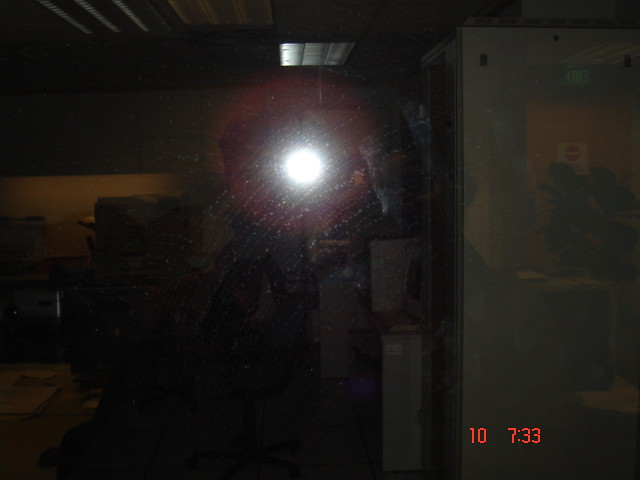The photograph appears to be taken inside a dimly lit warehouse or basement. Dominating the center of the image is a bright light that serves as the main focal point, casting stark shadows and creating a dramatic contrast with the surrounding darkness. In the lower right-hand corner, a sequence of orange digital numbers reads "10 7337:33," potentially indicating a date or a coded message, though its exact significance remains unclear.

To the right of the frame stands a tall, gray, reflective filing cabinet. The cabinet's surface mirrors a portion of the scene behind the photographer, including a wooden door adorned with a sign featuring a red prohibition symbol. In the upper left section of the image, a cluster of indistinct cabinets can be seen, but the details are obscured by the poor lighting and the intense brightness emanating from the central light source. The overall composition conveys a sense of mystery and ambiguity, with only a few discernible elements amidst the shadowy environment.